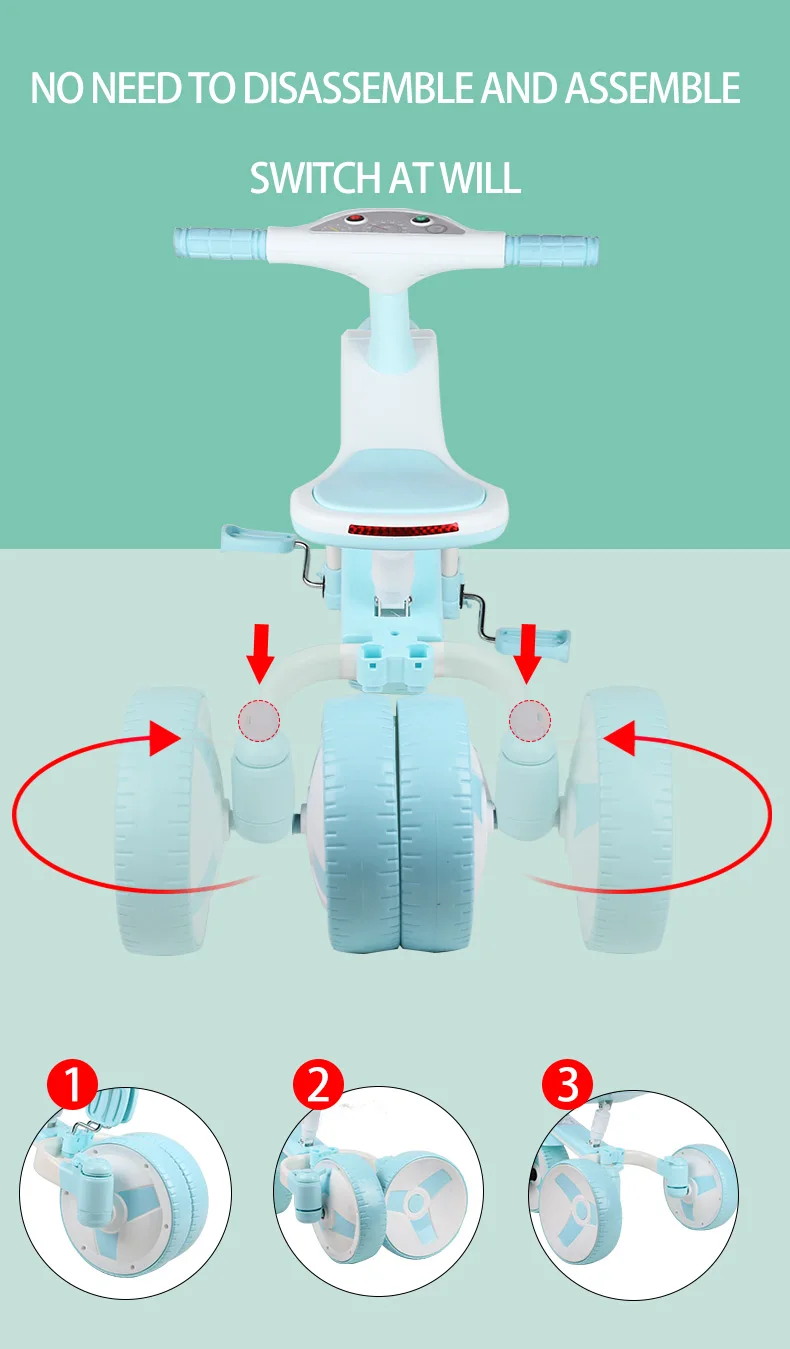Detailed Caption: 

The image showcases a light blue and white children's tricycle with an innovative design that offers adjustable configurations without the need for disassembly. Central to the image is the tricycle itself, surrounded by arrows that highlight the rotating and switching mechanisms of the four-wheel structure. Beneath the central tricycle, three detailed close-up images demonstrate the various wheel configurations and adjustment features. Although the overall presentation is sleek and minimalistic, a concern arises from the solid mint green background at the bottom half, as it causes the wheels to blend in and diminishes their visibility. Despite the minor issue with the background color, the clear, bold text and arrows effectively guide the viewer through the product’s functionalities. Overall, it’s a fascinating product with user-friendly design elements.